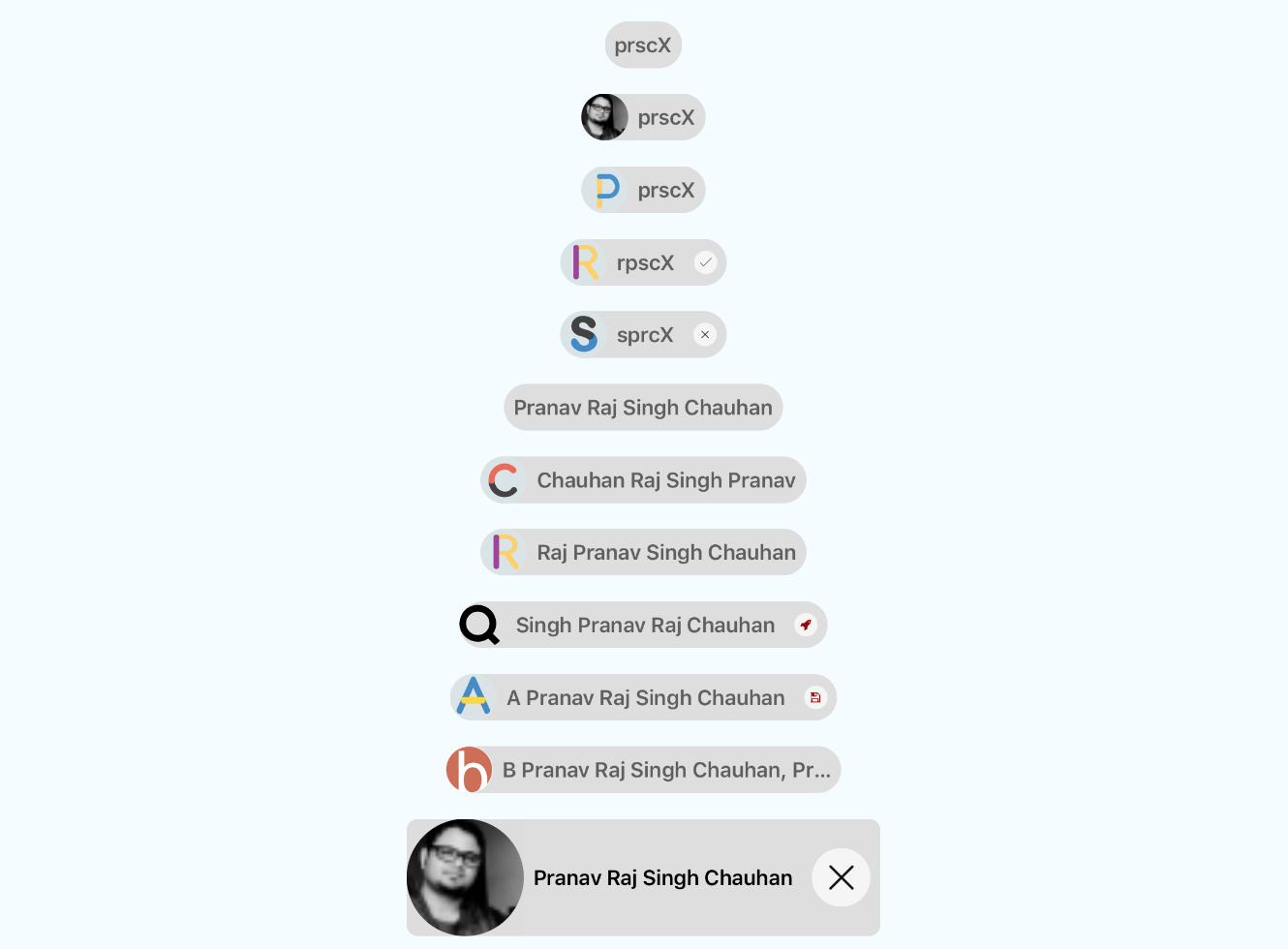At the top of the image, there is a gray, horizontally elongated oval with rounded edges. Inside this shape, the text "prscX" is written in lowercase letters, except for the uppercase "X." Below this, the oval widens slightly to display a black and white image of a person wearing glasses, alongside the repeated text "prscX."

Continuing downward, there is another oval of the same size, featuring the text "prscX" once more. This time, the letter "P" is highlighted in yellow and blue colors. Below this, the text reads "rpscX," with the "R" colored in purple and yellow.

Next, the text "sprcX" appears, with a large "S" colored in black and blue. Following this pattern, the subsequent oval contains the text "pranavchauhan." This text is repeated in several more ovals down the image.

Finally, at the very bottom, there is a much larger version of the earlier black and white image of a man with facial hair and glasses. Beside this enlarged image, the text "pranavchauhan" is displayed again.